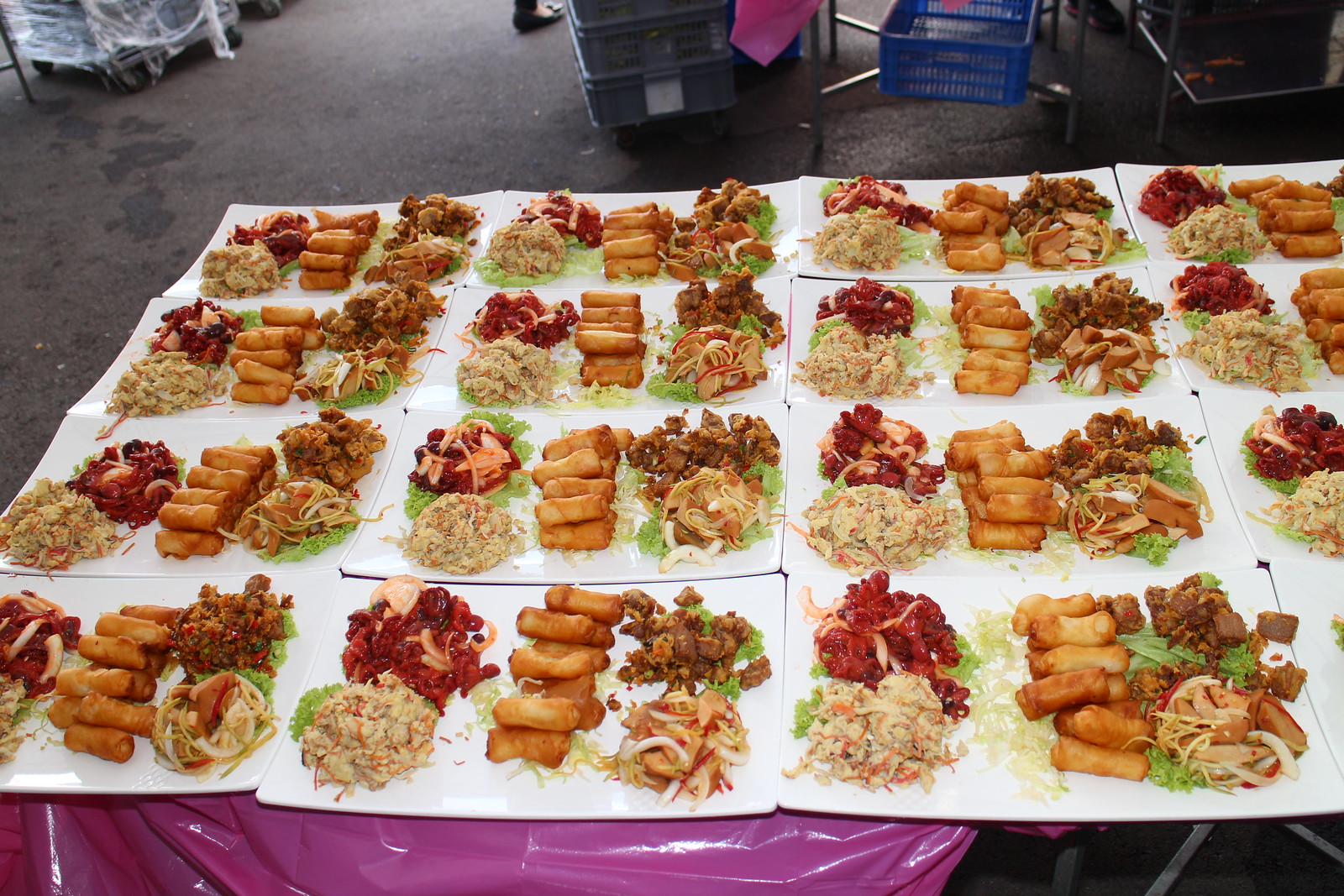This image captures a scene likely set in an open market or a catering hall with a dark concrete floor. A table covered in a shiny pink plastic tablecloth is prominently featured in the foreground. Arranged in a meticulous grid on this table are several rows and columns of white rectangular plates. Each plate contains five distinct types of food, including stacks of small oblong cylindrical brown egg rolls at the center, and garnished with parsley and shredded cabbage for an appealing presentation. Other foods on the plates possibly include different meats, fried rice, and coleslaw, all laid out on a bed of lettuce. Surrounding the table are various carts and portable tables holding gray and blue baskets or plastic crates. The table, which is supported by metal legs, appears to be situated on a wet or stained blacktop pavement.